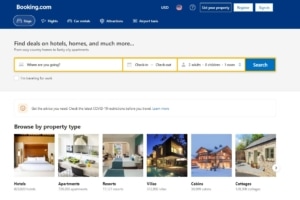The image captures a slightly blurry screenshot of a desktop computer screen displaying a webpage. At the top of the page is a wide horizontal blue banner with "booking.com" written in white text at the top-left corner. Directly below the banner are five distinct menu options. The main section of the webpage has a white background, featuring various smaller images related to accommodation options. Along the bottom, there are six smaller thumbnail images, each depicting different aspects of homes.

- The first image on the far left showcases a room with a white bed accompanied by two pillows, with brown and gold color tones.
- The second image depicts a breakfast nook, furnished with chairs and set around a white tabletop.
- The third image presents another bedroom setup, highlighting a bed adorned with white and blue bed sheets. The remaining images in the row are not described, but it's implied they continue representing various segments of home interiors or features.

Each image provides a visual glimpse into potential accommodations, aimed at users browsing for booking options on the "booking.com" website.